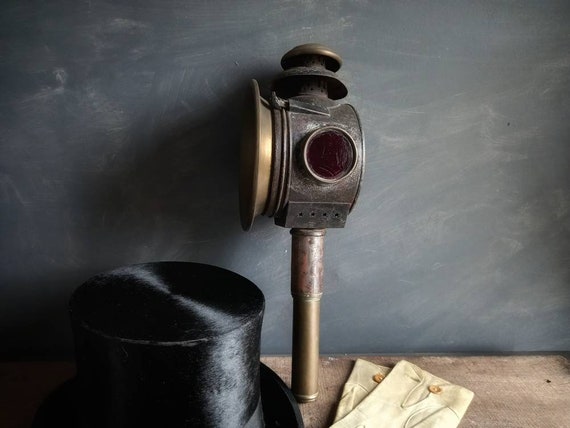This detailed image showcases a vintage device prominently placed in the center, composed predominantly of metal with varied textures and colors. The device comprises a goldish pole that ascends about a foot, supporting a blackish, cylindrical structure with patchy rectangular elements, rising an additional six inches. It features a conspicuous red circle at its center, accompanied by a gold, plate-like object extending from its left. The top of the device is adorned with two small circles. Adjacent to this antique apparatus, on its left, rests a black top hat, and to its right lie two small manila envelopes, possibly gloves with little yellow buttons. All these items are arranged on a light brown wooden surface, leaning against a nondescript gray wall.